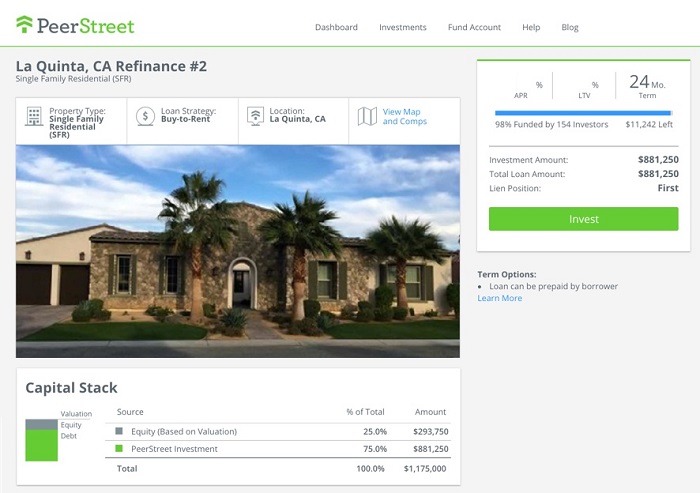The image displays a webpage from Peer Street, showcasing various navigation options such as Dashboard, Investments, Fund Account, Help, and Blog. Prominently featured on the webpage is a visual of a single-family residential home, along with detailed property information. The property is located in La Quinta, California, with a loan strategy specified as "buy to rent." Additional options include viewing a map and comparable properties.

At the top of the page, the header reads "La Quinta, California - Refinance No. 2," alongside key financial terms: APR percentage, Loan-to-Value (LTV) ratio, and a 24-month term. The investment opportunity is highlighted as being 98% funded by 154 investors, with only $11,242 remaining to reach the total investment amount of $881,250. The lien position is indicated as "First."

A prominent green "Invest" button is available for potential investors. At the bottom of the webpage, a capital stack section is displayed, using a green and gray bar to compare the investment distribution between Peer Street and Equity-Based funding. The breakdown shows that Peer Street contributed 75%, while Equity-Based funding accounts for 25%, together making up a total of $1,175,000.